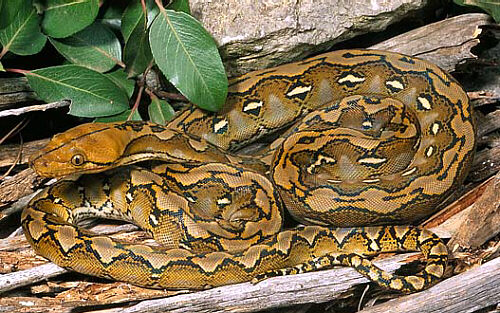The image showcases a beautifully coiled python resting among several wooden branches and logs. The snake features a caramel-colored head with striking brown eyes, facing the left side of the frame. Its body, predominantly golden-brown, is intricately patterned with black wave-like designs, black diamond shapes, and white lines, contributing to its effective camouflage against the wood. Green leaves hang from the top left corner, adding a touch of natural foliage to the scene, while a gray stone can be seen in the background. The python looks quite large, although its full length is obscured by its coiled position. The overall composition, with its mix of earthy tones and detailed patterns, highlights the python as a majestic yet subtly integrated part of its environment.